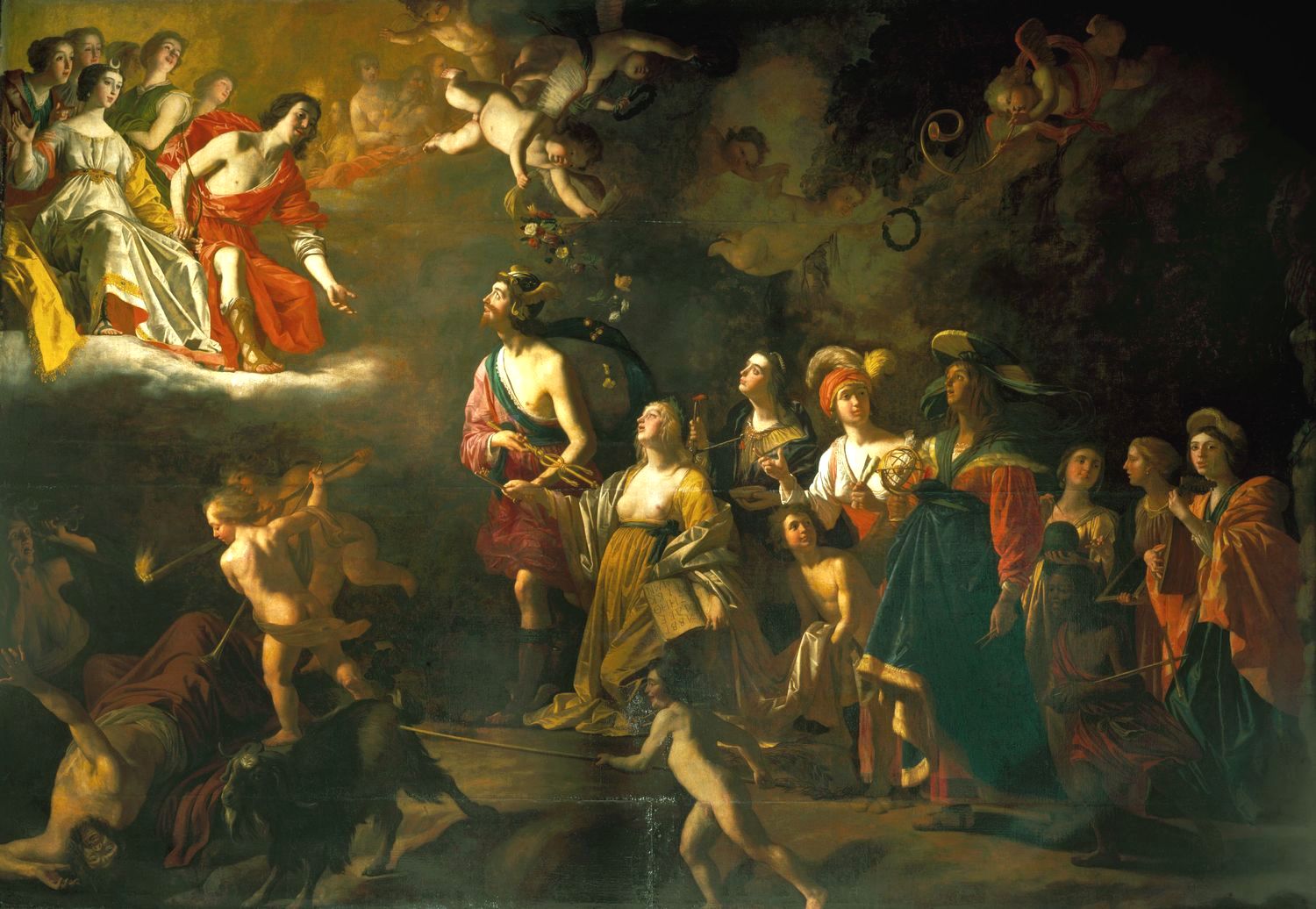This detailed Renaissance-style painting evokes a classical atmosphere, rich in symbolism and human emotion. The scene unfolds across a dynamic composition that interweaves earthly figures and celestial beings. In the upper left-hand corner, a group of six ethereal figures, possibly angels or deities, are seated on a cloud, watching over the events below. Among them is a prominent woman wearing a U-shaped crown, suggestive of her elevated status. The central figure, a woman adorned in a gold dress, is being held by a horned man dressed in a robe, his gesture pointing a pronged fork towards her, adding an element of tension.

The lower right quadrant is populated by a diverse array of individuals clad in flowing, old-fashioned gowns and large hats. One notable figure is a bare-chested woman, symbolizing vulnerability. This group of people directs their gaze and gestures upward towards the celestial beings. On the right, a spectrum of colors including green, brown, white, and red highlights the vividness of the scene.

Down in the lower left quadrant, the dynamic shifts as cherubic figures armed with prongs are seen attacking a fallen man and a terrified woman, adding a dramatic layer of conflict. In the forefront, another figure seems engaged with a wheelbarrow or possibly dealing with a large bull on wheels, further enriching the multi-layered narrative. The painting encapsulates a biblical or mythological tableau, blending human struggle with divine oversight, creating a rich tapestry of emotion and action.